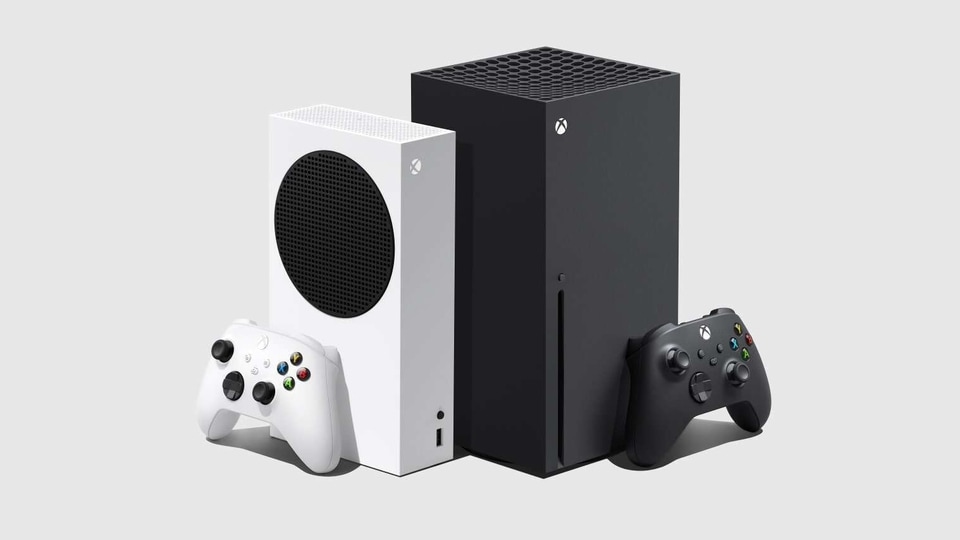This photograph showcases a modern and detailed comparison of two Xbox gaming systems, placed side by side against a gray background. On the left, the smaller, slimmer, white Xbox Series S stands upright, featuring a prominent round black vent on its side. Accompanying it is a matching white wireless controller resting against the console, identifiable by the distinctive "X" logo in the upper left corner. On the right, the larger, square-shaped black Xbox Series X is displayed, recognizable by its top vent and front disc drive slot. A corresponding black controller leans against this console, also bearing the "X" logo, visually confirming their association. The image emphasizes the differences in size and design between the older and newer Xbox models.